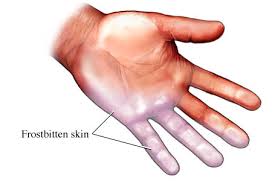The image is a detailed medical diagram depicting an open male hand with parts affected by frostbite. The hand is oriented with the palm facing up, angled slightly down and to the right. On the left side of the image, the term "frostbitten skin" is prominently labeled, with lines pointing to various frostbitten areas on the hand. Specifically, the pinky finger and parts of the inner palm are highlighted with a chalky white discoloration. Other parts of the hand exhibit varying degrees of frostbite, including the first two fingers and the tips of the next two fingers, which show a whitish-blue and purple hue indicative of frostbite damage. The remaining areas, including the thumb and lower sections of the second set of fingers, are mostly unaffected, maintaining a natural tan color. This comprehensive diagram serves to clearly demarcate the progression and affected areas of frostbite on the hand.